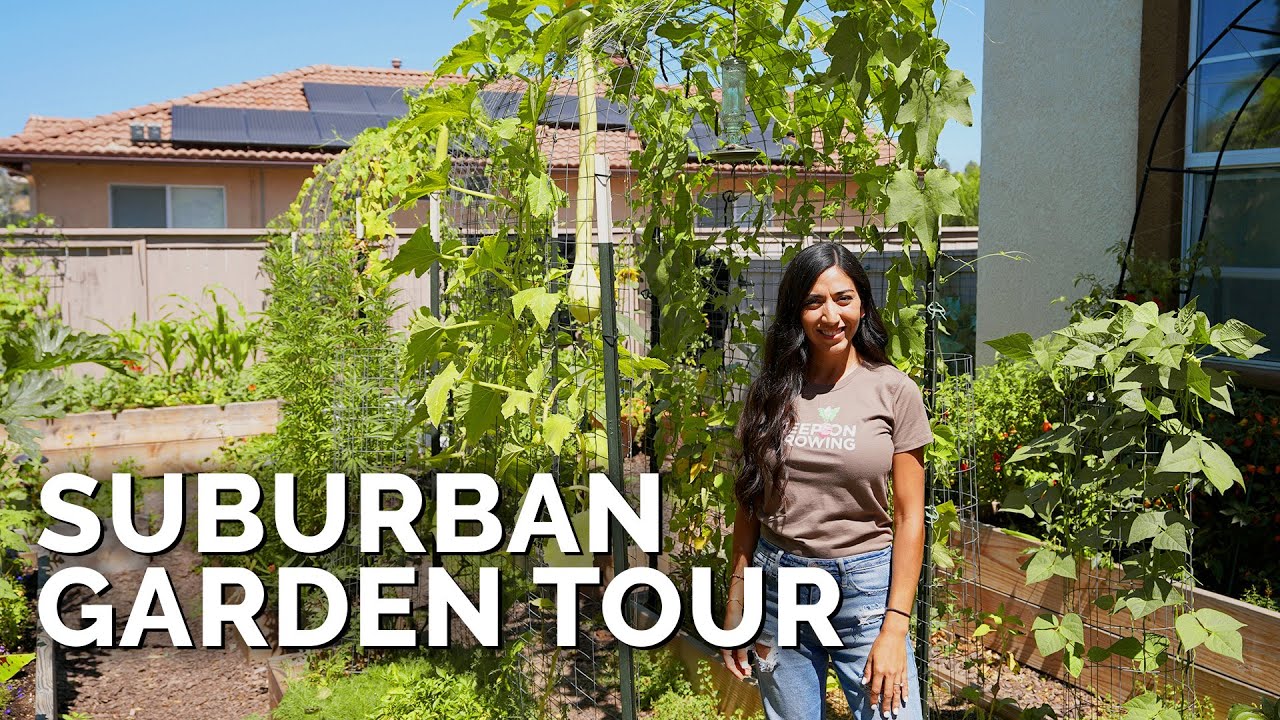In the image, bold white font in capital thick letters prominently states "SUBURBAN GARDEN TOUR." Positioned in the middle of the picture is a woman standing in the garden, framed against a backdrop featuring a light brown house with red roofing tiles and solar panels. The house is bordered by a light brown fence, bringing a suburban charm to the whole scene. The woman is dressed in blue jeans and a gray shirt emblazoned with the word "growing" and other unreadable text. She has a warm smile on her face, though she is squinting slightly due to the bright sunlight shining directly at her. Her long, dark brown hair flows down to her waist, with half of it cascading over her shoulder. Surrounding her are an array of lush plants, vines, and plant beds that reach up to her height, vividly capturing the vitality of the suburban garden. Suspended above the scene is a clear blue sky, encapsulating the serene and inviting atmosphere of the garden tour.